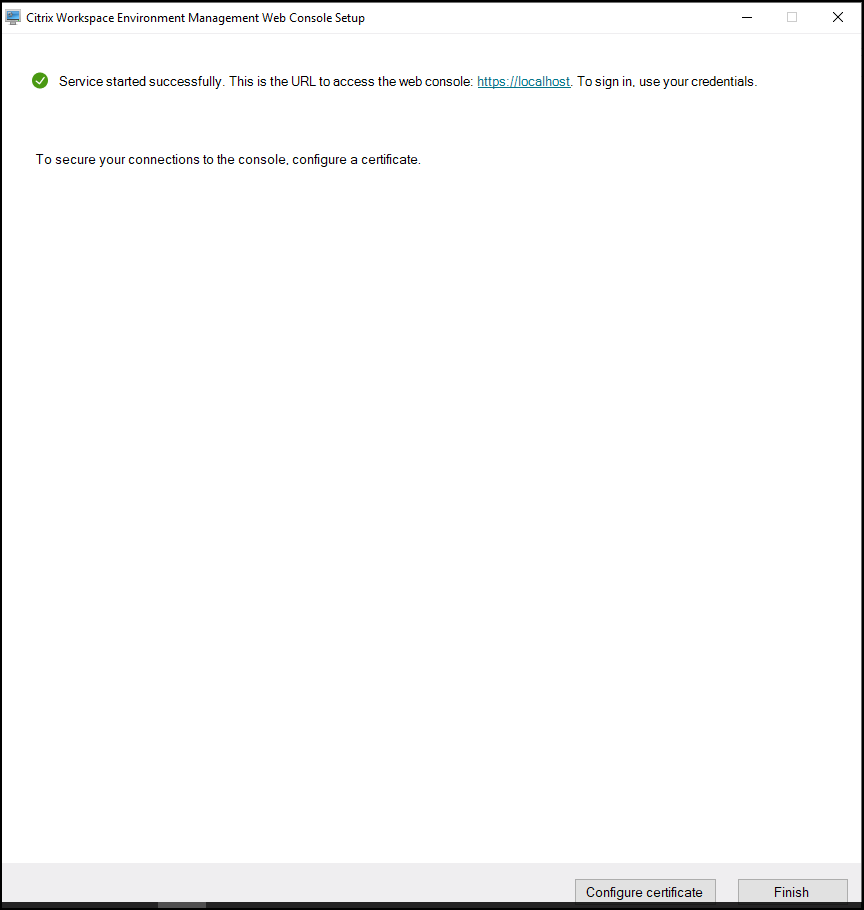The image displays the setup page for the Citrix Workspace Environment Management web console. Key text elements present on the page include confirmation that the service has started successfully. Users are directed to access the web console via the provided URL: https://localhost, depicted as a hyperlink. Instructions indicate that users should sign in using their credentials. Additionally, it is recommended to configure a certificate to secure connections to the console. 

At the top right corner of the image, there are minimize and close buttons. The bottom right corner features options labeled "Configure Certificates" and "Finish."